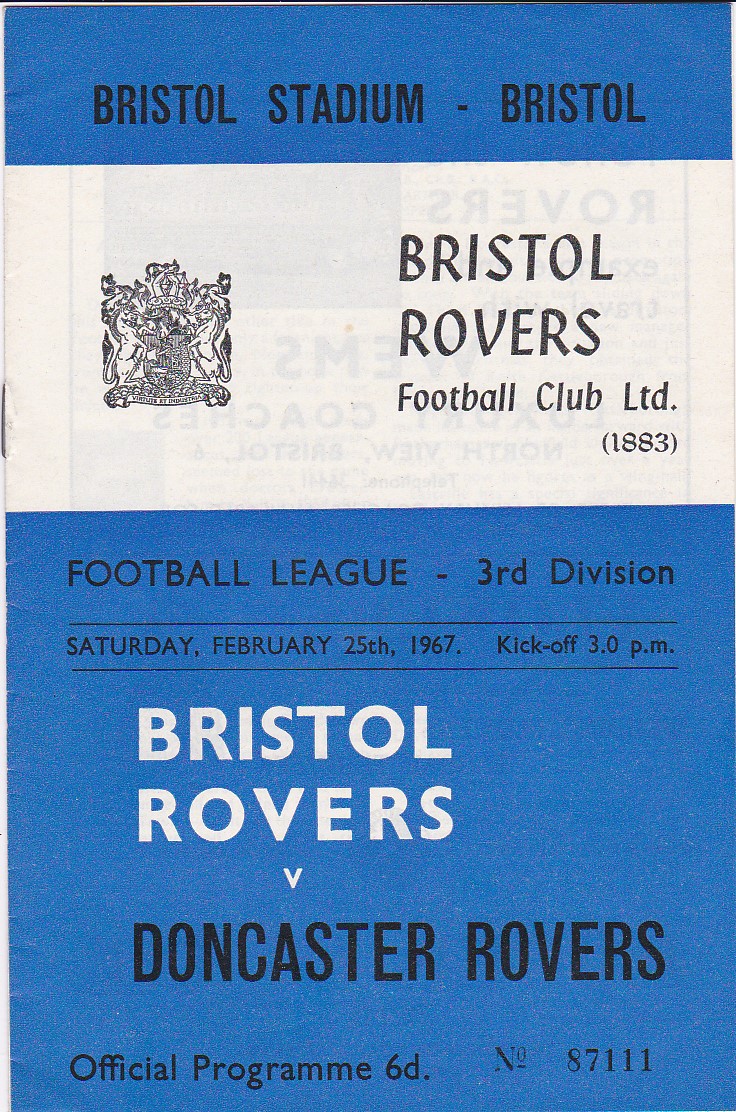The front page of the Bristol Rovers football program features a striking vintage design with predominant blue and white colors. At the very top, a blue horizontal band spans across the cover with bold black text reading "BRISTOL STADIUM - BRISTOL". Below this, a prominent white section showcases the club's emblem on the left, depicting an intricate logo with a shield, flanked by black text on the right that reads "BRISTOL ROVERS FOOTBALL CLUB LIMITED (1883)". The lower half of the cover returns to solid blue, beginning with black text that states "FOOTBALL LEAGUE - 3RD DIVISION" and "Saturday, February 25th, 1967. Kickoff 3.00 p.m.". Further down, in white letters, it features "BRISTOL ROVERS" followed by "v. Doncaster Rovers" in black. At the very bottom, it notes "OFFICIAL PROGRAMME 6D" alongside the program number "87111".